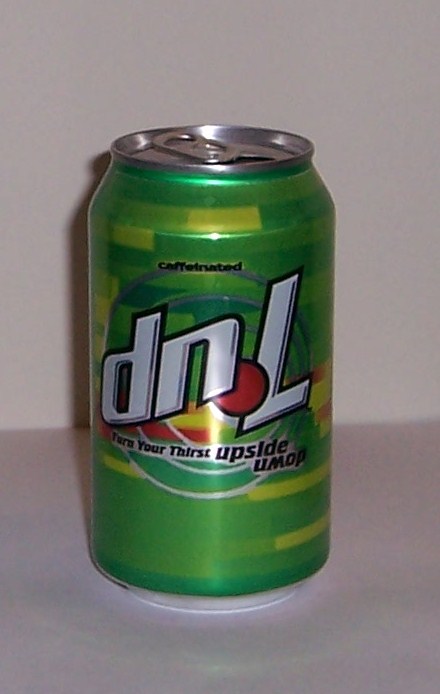This detailed photograph captures a close-up view of a 7-Up can set against a background that, due to the photo's color rendering, appears to be light lilac, both on the countertop and the backdrop. The 7-Up can itself is a traditional green aluminum can with a silver top, featuring an unopened pull tab. Uniquely, the text "7 Up" is presented upside down, accompanied by the word "caffeinated" (though this is somewhat difficult to read clearly). The "7 Up" text is in white and includes a depiction of a cherry. Below this, the phrase "Turn your thirst upside down" is displayed, associated with an assortment of green circles and lighter green and yellow rectangular shapes, adding dynamic elements to the design.